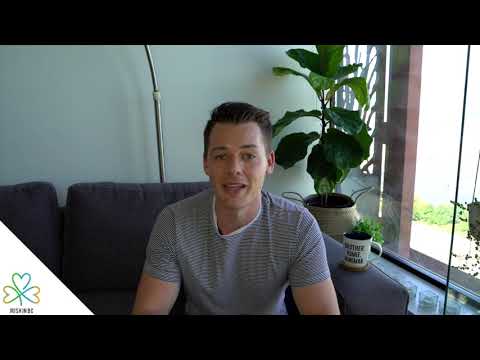In this image, a Caucasian man with a short buzz cut and neatly combed back hair sits on a dark gray couch, centered in the frame. He is wearing a light gray shirt with very fine stripes and appears to be mid-sentence, smiling and looking directly at the camera. To his right, on the arm of the couch, rests a white coffee cup with blurred black text, placed on a coaster. Further to the right, a lush green plant with large leaves is positioned near a window, through which you can see greenery and a wooden post outside. Behind the man is a white wall. In the bottom left corner of the image is a shamrock logo, designed with three heart-shaped leaves, accompanied by some blurred text. The overall scene suggests a casual, home setting, possibly during a video call or recording, and is characterized by colors including shades of gray, green, and white. The image quality is low, with visible compression artifacts and horizontal black bars at the top and bottom, contributing to its reduced clarity.